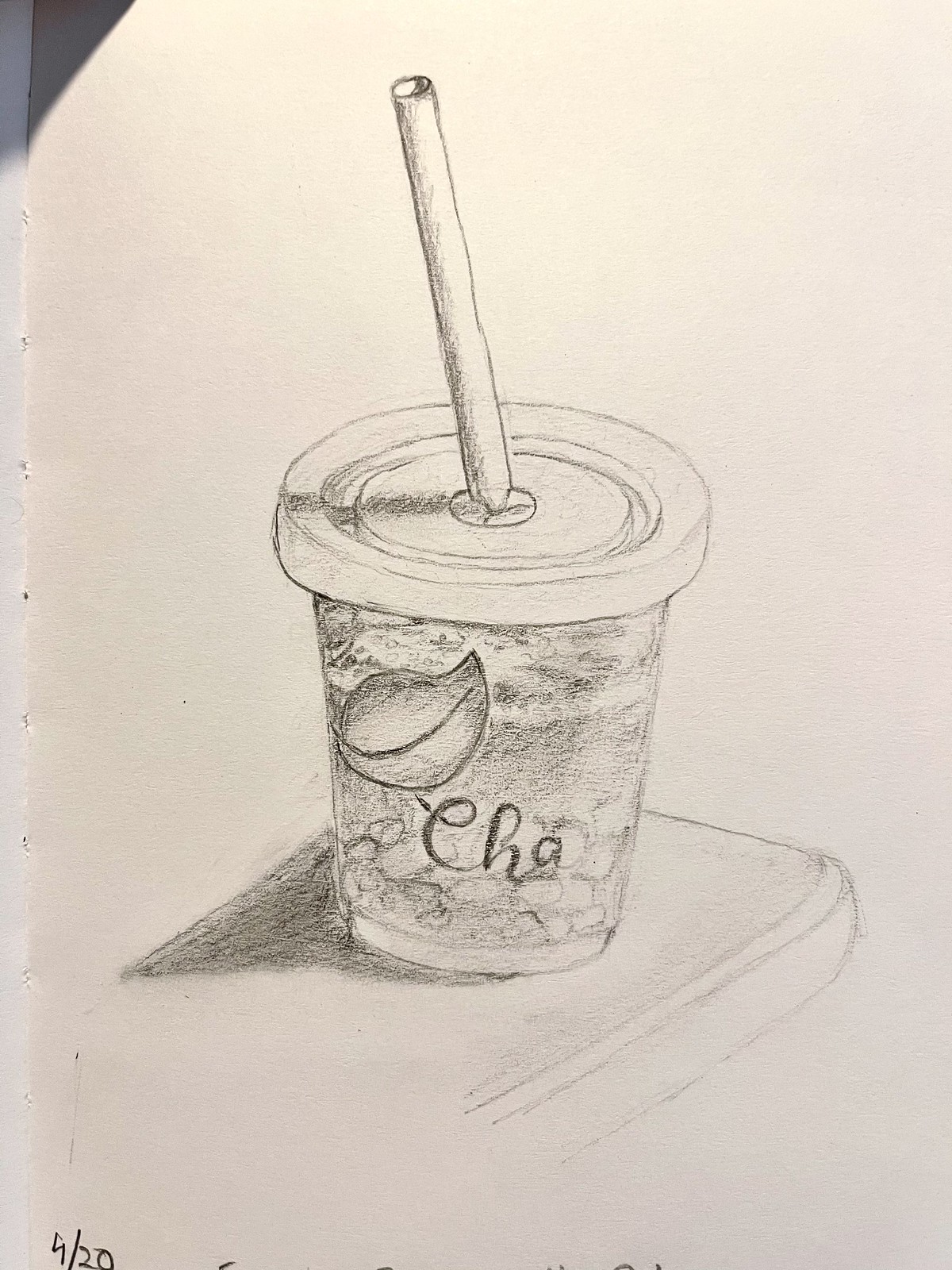A meticulously penciled illustration depicts a small fountain soda cup perched delicately atop the armrest of an armchair. The cup, complete with a lid featuring a central opening for the straw, exudes a quaint charm. The straw itself is slightly tilted towards the left, adding a touch of realism to the scene. Adorning the cup is a detailed drawing of a leaf, symbolizing perhaps an eco-friendly or organic beverage, with the partial inscription "ch a" visible at the bottom. The overall composition and careful attention to detail suggest a thoughtful and artistic touch in this quaint, everyday scene.